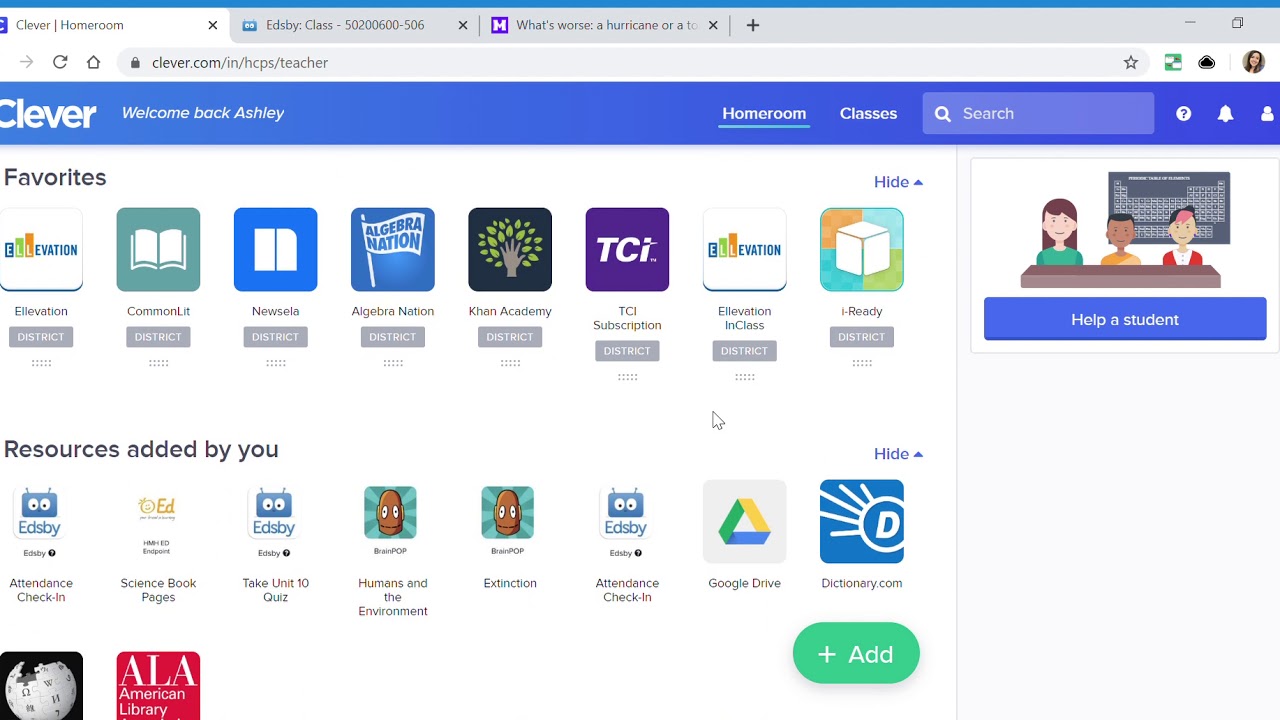This horizontal image, likely a screenshot from a computer screen, features a predominantly white background. At the very top of the image is a thin, cerulean blue line that spans the width of the screen, indicating the active window border. Below this line, several browser tabs are visible, with "Clever Homeroom" being the currently selected tab. Other open tabs include "Edsbee class" and a partially visible tab that likely says "Hurricane Aura tour." There is also a plus sign for adding new tabs.

On the right-hand side of the window, the minimize, maximize, and close buttons are located, while the forward navigation button is also present. On the left-hand side, there are buttons for refreshing the page and navigating to the home page, along with a gray search bar displaying the URL "clever.com/in/hcps/teacher." To the right of this search bar, there is a star icon used for bookmarking, additional icons, and the user's profile picture which features a lady.

Below the browser interface is a long blue rectangular box with the word "Clever" written in white, followed by the text "Welcome back, Ashley." Next to this, there are menu options with "Homeroom" underlined, indicating the active section, and tabs labeled "Classes" along with a search bar, question mark icon, bell icon, and person icon.

The main content area is divided into sections. First, there are favorites, which are displayed as small squares with pictures and names of various apps. Following this, there is a "District" section with a grid of resources provided by the district. Below that, there is a section titled "Resources added by you," showcasing the user's personal additions. A green button labeled "Add" is also present for adding more resources.

On the right-hand side of the content area, there is an image of a group of students seated at a desk with a chalkboard behind them. Adjacent to this image is a blue button labeled "Help a student."